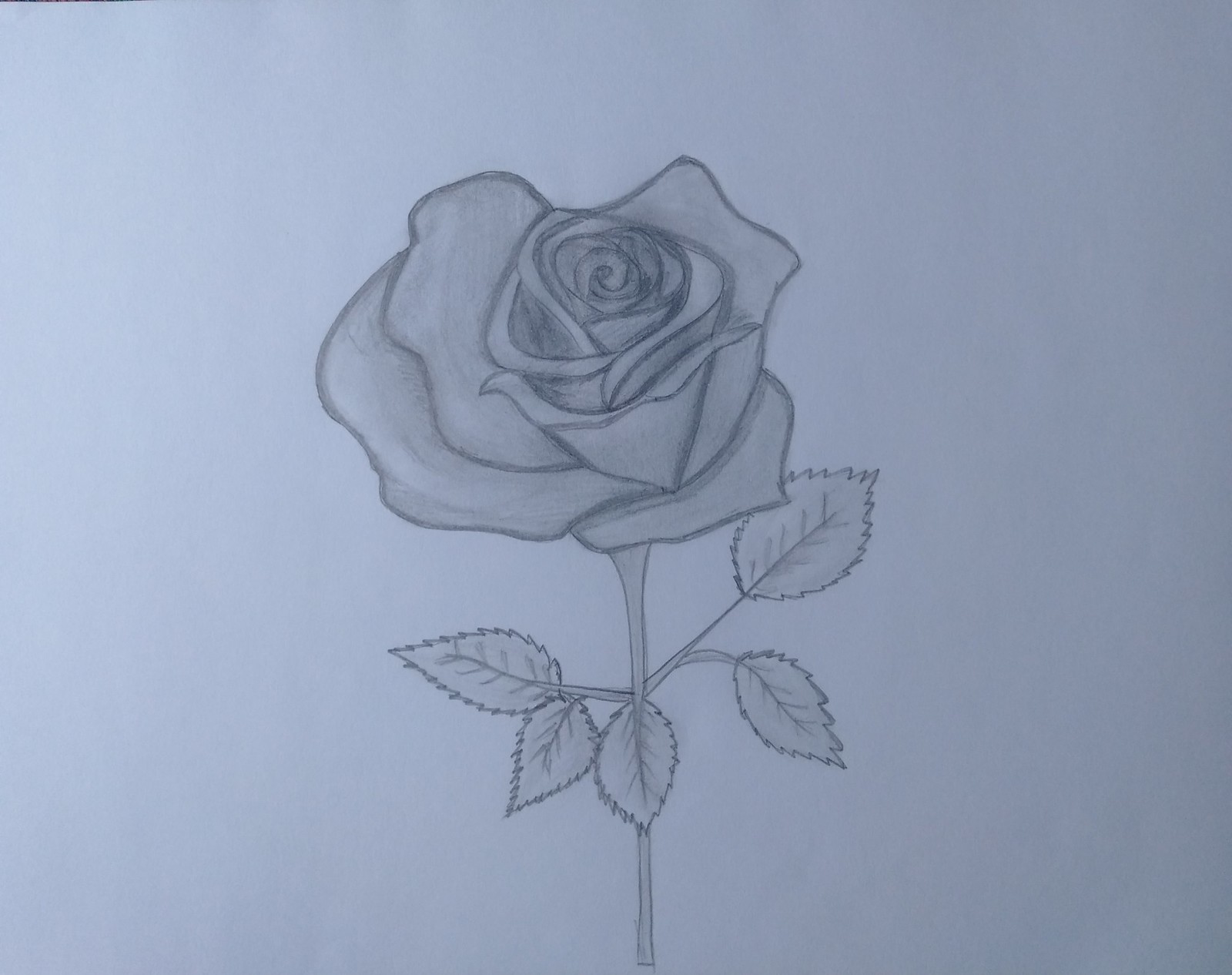This is a highly detailed pencil sketch of a rose drawn on a blank white piece of paper. The rose itself is intricately shaded, with its petals rendered in varying shades of gray, becoming darker and nearly black towards the tightly curled center. There are five leaves surrounding the rose, each adorned with fine, jagged edges and detailed vein structures. The leaves on the left side are noticeably smaller than those on the right, with the largest leaf oriented towards the right corner of the image. The delicate leaves and stems are captured with meticulous detail, demonstrating proficient use of shading to create depth and texture. The overall composition is clean, with no visible defects or elements other than the rose and its leaves, making for a striking black-and-white artwork.